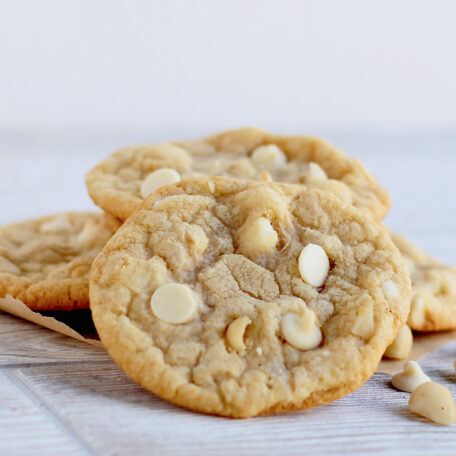The image features a stack of four round, flat cookies on a light wood-grain surface, possibly tile, with a blurry white background. These light brown cookies contain white chocolate chips and macadamia nuts. They rest on brown parchment paper. One cookie leans forward, fully exposing its top, while three are stacked behind it. Scattered around are a few loose white chocolate chips and a macadamia nut piece on the lower right side, adding to the detail of the scene. The cookies show a slightly darker bake along the edges, highlighting their texture.